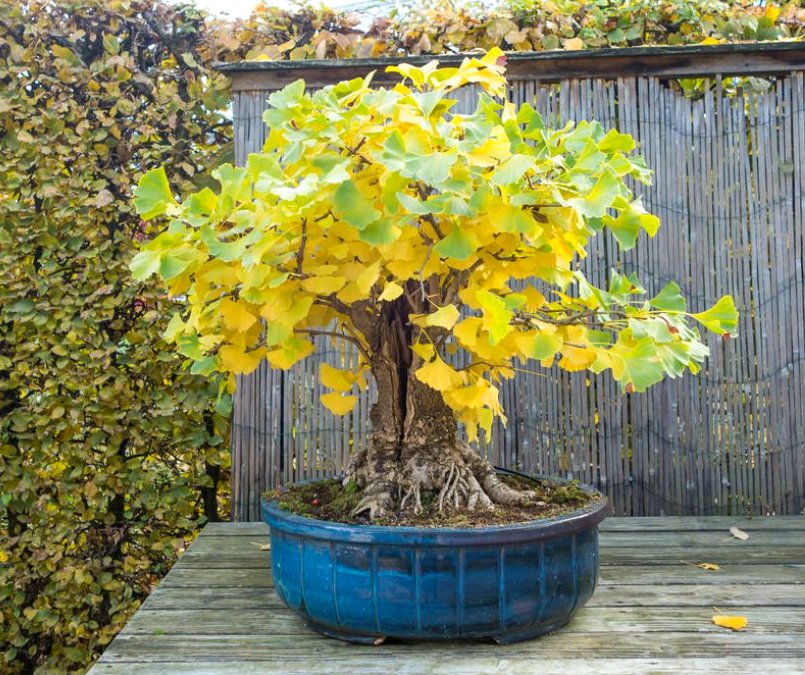This captivating image showcases a mature bonsai tree housed in a charming blue pot that fits it perfectly, neither too wide nor too shallow. The trunk of the bonsai tree appears robust, indicating its advanced age. The foliage is a beautiful blend of green and yellow hues, suggesting excellent care and meticulous attention. Bonsai trees are known for their finicky nature and sensitivity to environmental changes, making this healthy specimen a testament to the owner's dedication and skill in bonsai cultivation.